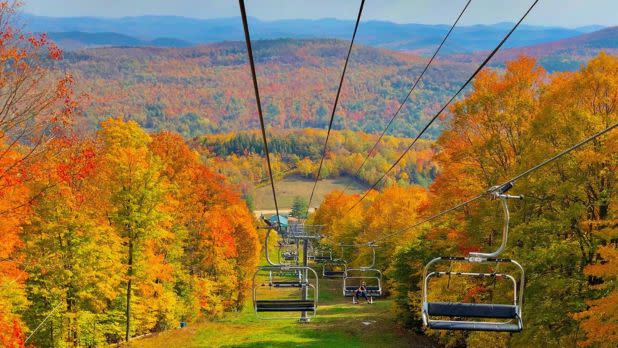The image captures a scenic outdoor setting during autumn, featuring a vibrant display of trees adorned with leaves in stunning shades of orange, yellow, red, and hints of green. Central to the image is a series of five cables stretching from the top to the background, suggesting a ski lift or monorail system equipped with metal cable cars, which appear black in color. Some of these cars are empty, while one potentially carries a blurry, indistinguishable figure. These cable cars hang over a grassy pathway flanked by trees on both sides, their foliage accentuating the fall aesthetic. In the distance, the landscape unfolds into a series of hills and mountains, painted in muted autumnal hues, beneath a sky that transitions from a cloudy hue at the horizon to a clearer blue overhead. The scene combines both natural beauty and recreational infrastructure, creating an inviting atmosphere for onlookers or visitors.